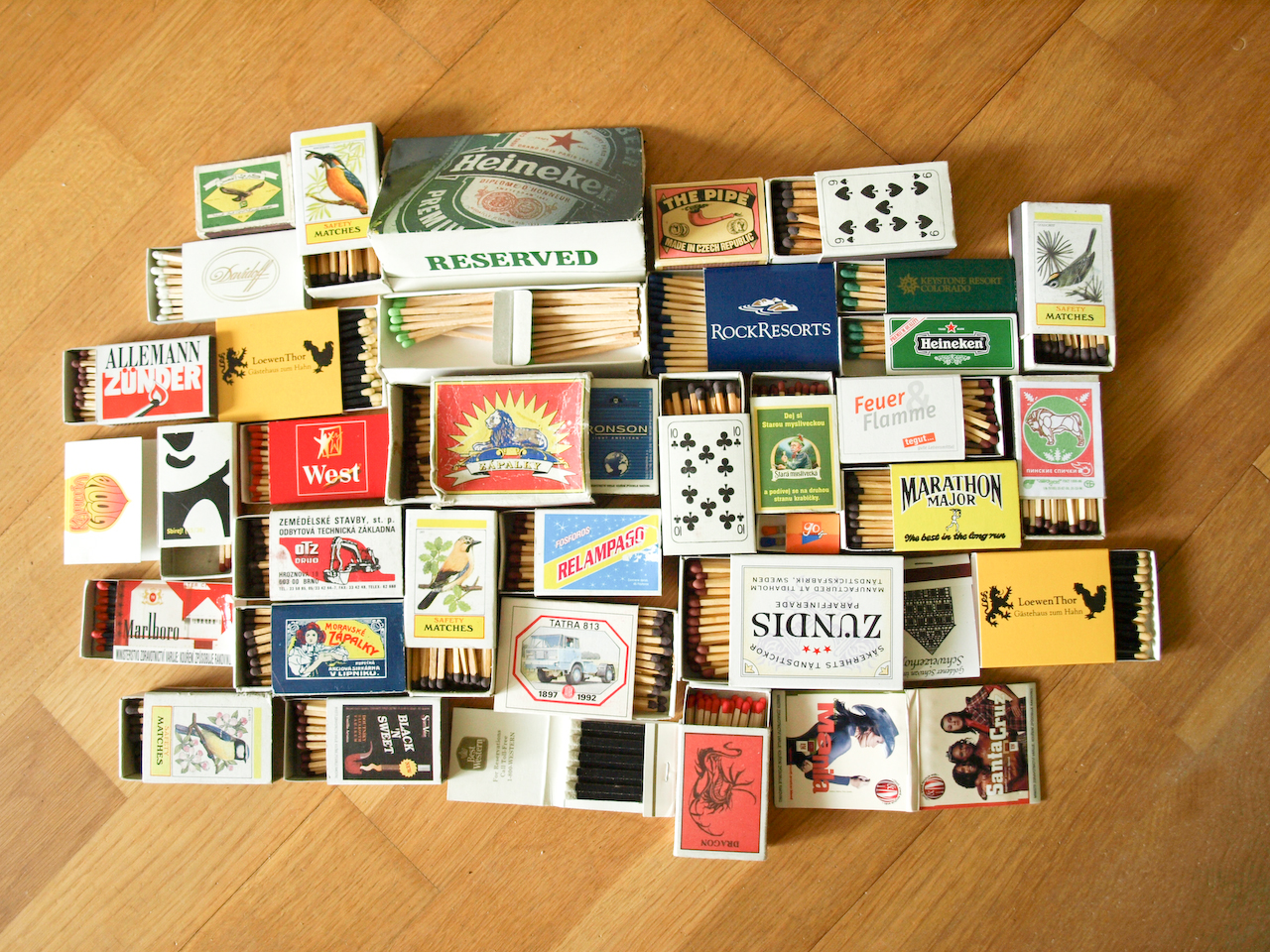This photograph captures a meticulously arranged collection of unique matchbooks sprawled across a reddish-golden hardwood floor. The collection features a diverse array of over 15 visually distinct matchbooks, each partially open to reveal the matches within. The matchbooks exhibit various striking tip colors and display a wide range of branding. Among the identifiable brands are Heineken, with one matchbook even repeated, Marlboro, West, The Pipe, Marathon Major, Rock Resorts, Alamond Thunder, Red Lampa, and Zundes. Notably, other matchbooks showcase designs like a spade poker card, adding to the collection's eclectic and colorful nature. The matchbooks differ in size and design, reflecting a rich tapestry of potentially both familiar and unfamiliar brands.